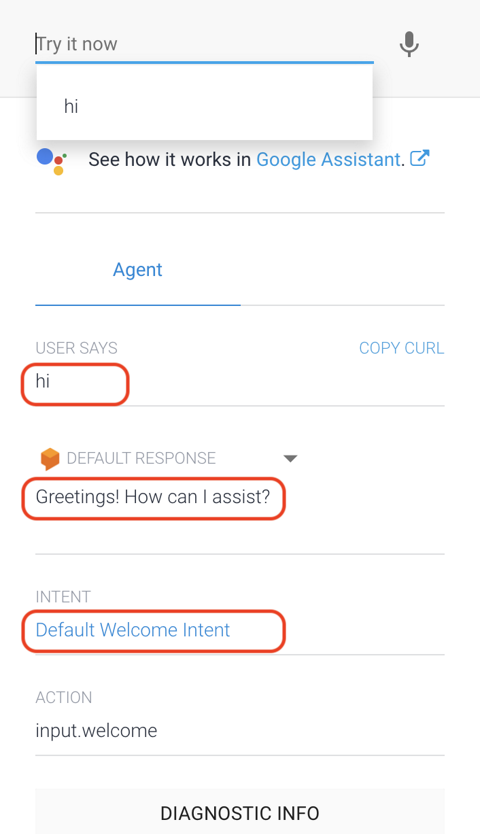The image showcases an interface for Google Assistant on the Google platform. In the upper top left corner, we see a prompt that says "Try it now," with a cursor positioned before the 'T'. Below that, a white dropdown box with a blue line at the top displays the word "Hi." This is part of the "Agent" tab, which is highlighted in blue with a corresponding blue underline.

Further down, next to "User says," the word "Hi" is circled in a red box. Beneath this, there is a section labeled "Default response" with a dropdown arrow. Within this, text in a red box reads "Greetings! How can I assist you?"

At the bottom of the interface, there's a row labeled "Intent," with the phrase "Default Welcome Intent" written in blue text and surrounded by a red box.